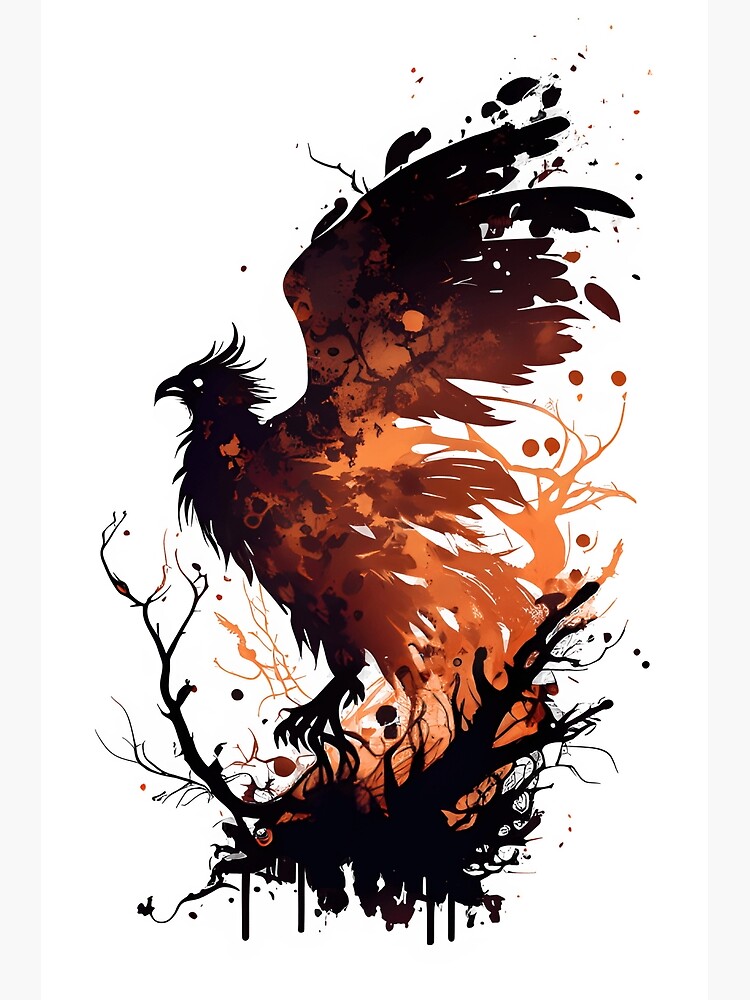The image features a detailed and striking depiction of a phoenix rising from the ashes, set against a white background with a gray border. The phoenix, a majestic bird, occupies the center of the composition. It is an artwork that intricately combines digital painting with elements reminiscent of graphic design and ink drawing. The bird is surrounded by swirling flames and dark, contorted branches that root it to the base of the image. 

The phoenix's head and upper wings are predominantly black, contrasted sharply by its white eyes and a sharp, black beak. The middle part of the bird transitions into vibrant hues of orange and burnt orange, with splashes of lighter and darker shades, giving the impression of it emerging from the intense fire below. The lower body and tail feathers blend into the brown and orange flames, which are rising upward.

Curvy black branches and stems with dripping black lines form the base where the phoenix is perched. These branches starkly contrast with the orange flames, enhancing the dramatic effect of the bird soaring from the fire. The wings, both expansive and tall, are depicted in a dynamic motion, appearing to flap upward. Feather-like elements and black splatters extend from the wings, adding to the abstract and vivid portrayal of the scene. 

Overall, the image exudes a sense of rebirth and triumph, capturing the essence of the phoenix legend perfectly.